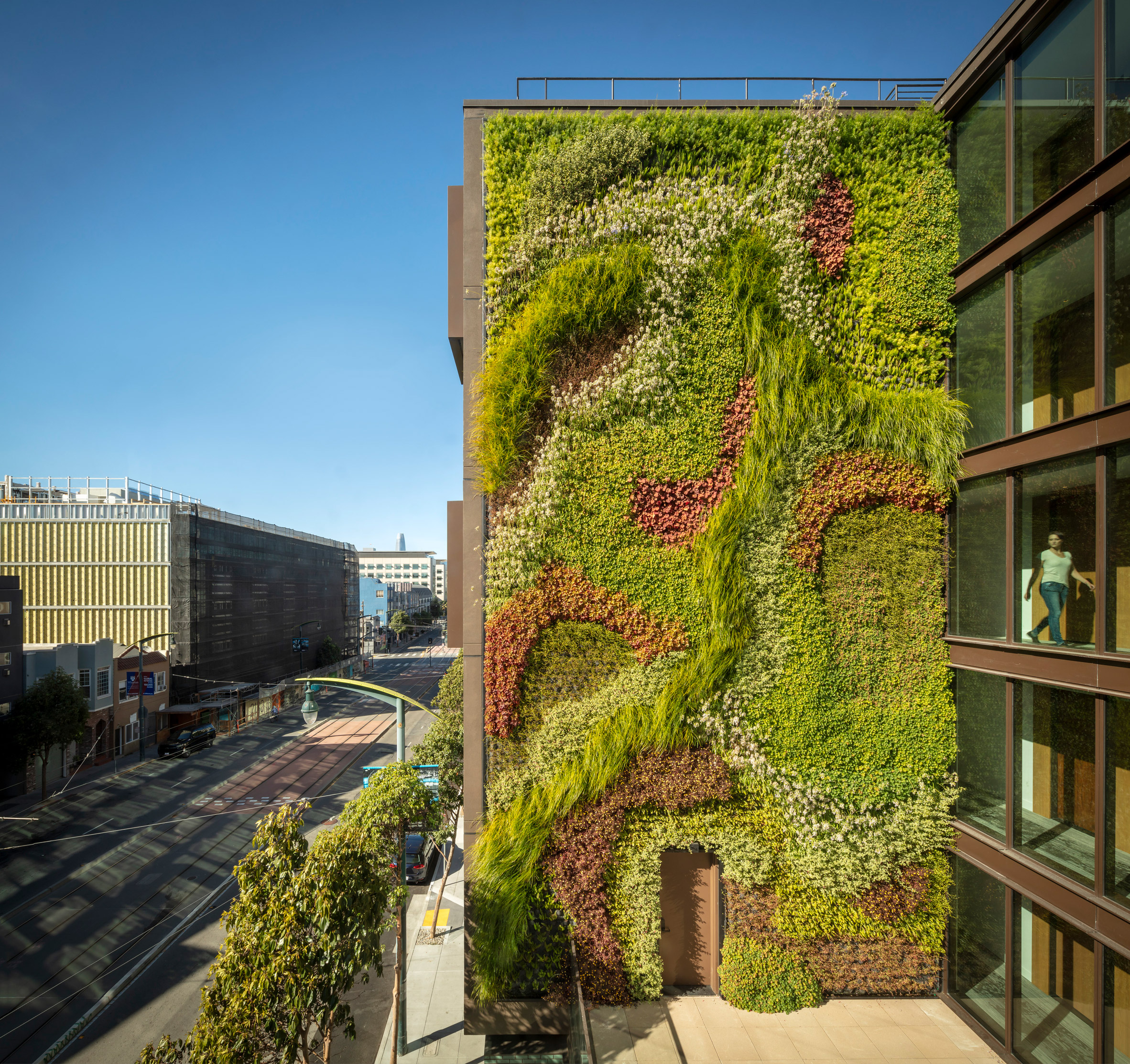This striking image captures a unique greenscaped wall adjacent to a modern five-story office building with all-glass exterior windows. The living wall, reminiscent of city greenscaping techniques, is covered in various types of flowering grasses and mosses, creating a rich tapestry of textures and shades of green, punctuated by patches of brown and white. The grasses grow in abstract forms and diverse lengths, interspersed with small wildflowers, including white and possibly red clovers, contributing to its vibrant, almost artistic appearance. At the very bottom of the wall, a small door adds an unexpected element to the scene.

On the third floor of the building, a woman in a white tank top and blue jeans can be seen walking towards the camera, turning her head as if to admire the lush vertical garden. The street below the wall is empty, bordered by trees and a larger building, all beneath a clear, blue sky devoid of clouds. This image beautifully juxtaposes urban infrastructure with nature, creating a serene, visually captivating urban oasis.